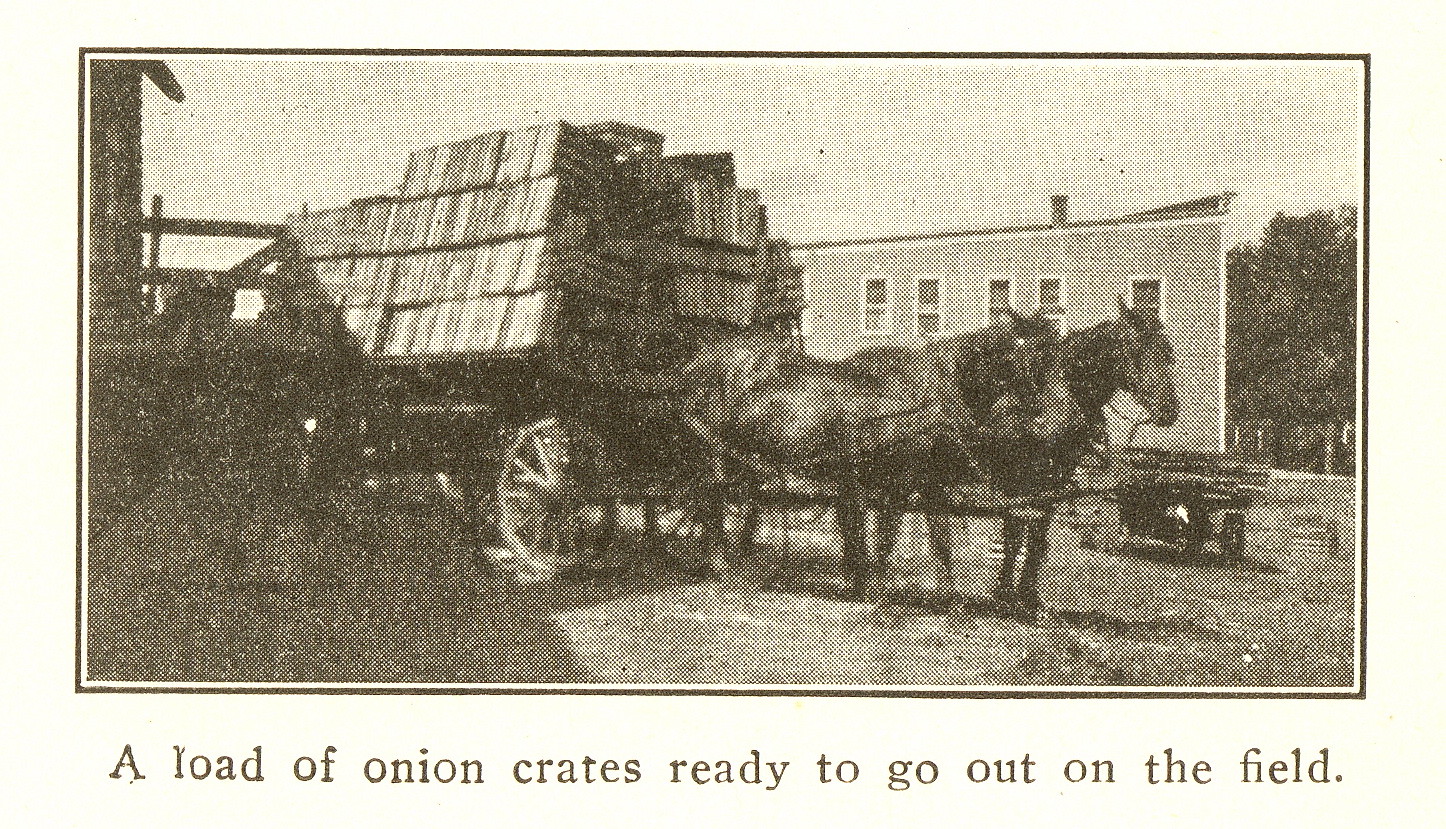This weathered black and white photograph captures an era gone by. It features a horse-drawn carriage loaded with numerous, seemingly heavy crates, ready to transport their bountiful load of onions to the field. The image prominently displays two horses standing steadfast and poised to pull the overloaded wagon. Surrounding the scene, one can discern a building—perhaps part of a barn—and several trees in the background, adding depth and context to the setting. A patch of grass lies just to the right of the horses, where an ambiguous object rests. Additionally, bits of hay are scattered in the scene, enhancing the rustic, agricultural atmosphere. The photograph is horizontally oriented, and a caption beneath reads: "A load of onion crates ready to go out on the field."